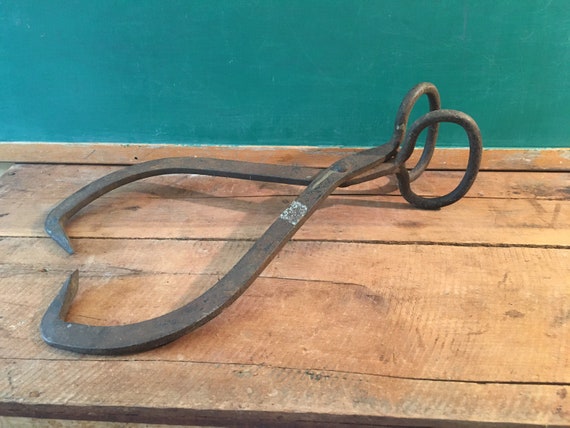The image depicts a vintage ice block tong placed on a rustic, wide-planked wooden table or bench against a medium blue or turquoise wall. The dark, weathered metal tool features large handles connected by a hinge, with the metal extending outward before curving back into two sharp, medium-length spikes designed to pierce and lift blocks of ice. Although there is a remnant of a torn-off label or perhaps faded white paint on the tool, it otherwise shows its age and wear prominently. The setting and condition of both the tool and the surface it rests upon invoke a sense of historical utility, possibly linked to an old ice shack or similar setting where such tools were once essential for handling large ice blocks.